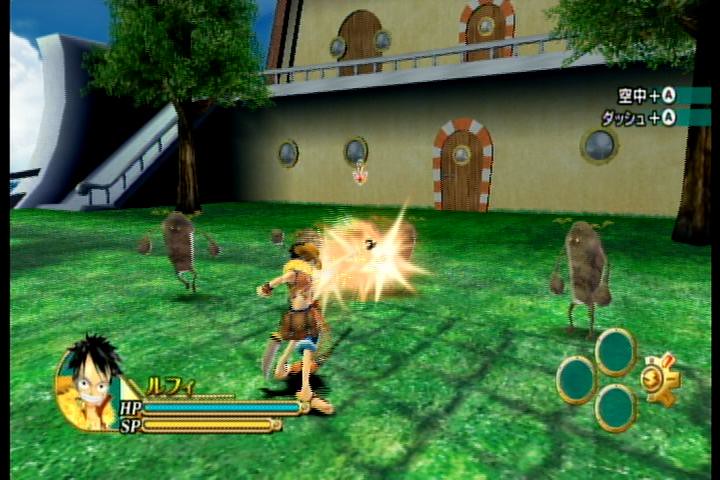Screenshot from a Japanese RPG game showing the hero in combat against three distinct enemies. The scene is set on a vibrant green grassy terrain. In the background looms a two-story building featuring a door on each floor. The bottom level showcases three porthole windows, and there's a peculiar staircase resembling a slide leading to the second floor. The backdrop includes two visible trees, a clear blue sky in the top left corner, and a lone white cloud. The foreground displays the user interface, with a meter indicating HP and SP levels, a character portrait, and accompanying Japanese text.